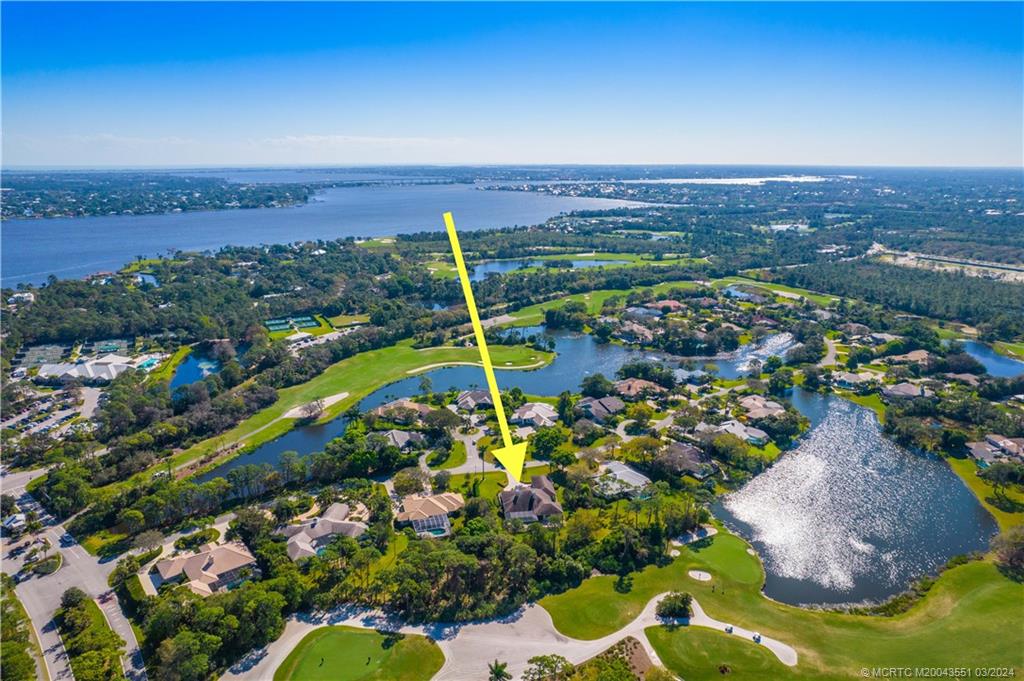This aerial image captures a picturesque waterfront neighborhood, possibly located in an exotic locale such as Hawaii. The neighborhood features an array of tan and white roofed bungalows, neatly arranged within a cul-de-sac layout. A large yellow arrow prominently points to the fourth house in from the left, drawing specific attention to it. The area is rich with lush greenery, including trees, bushes, and vibrant green grass, gracefully interspersed among the houses. Meandering inlets of dark blue water intricately weave throughout the neighborhood, leading out to a greater bay area. In the bottom right corner, a golf course can be spotted, adding to the area's charm. The backdrop is framed by the horizon, where strips of land meet a stunning ocean, beneath a sky that transitions from a lighter blue to a deeper hue. The image carries a copyright notice at the bottom right reading "MCRTC," along with additional letters and numbers, and is dated March 2024.